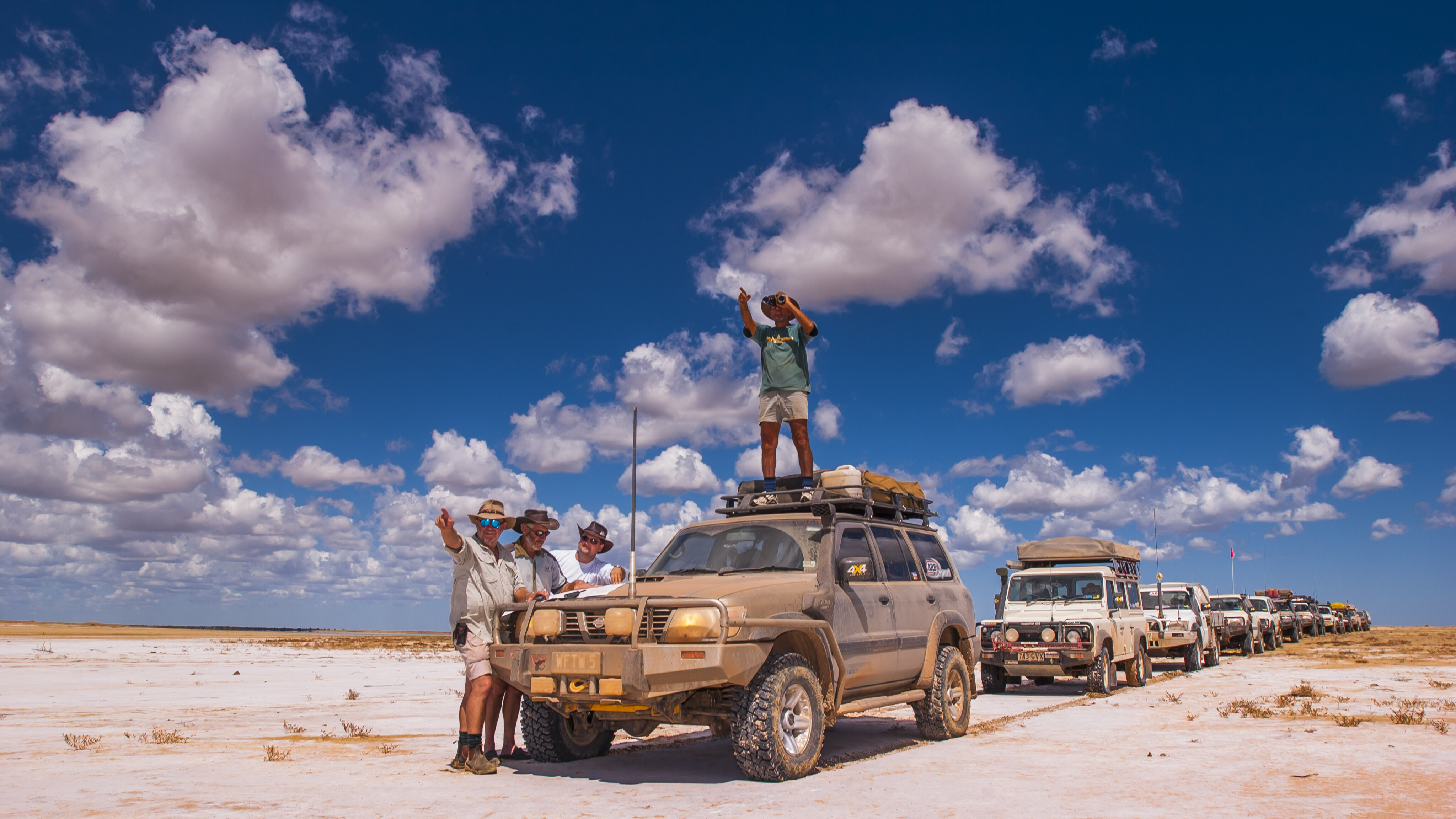In this photo set in a desert-like terrain with a sandy, white ground dotted with patches of greenery and weeds, a convoy of eleven off-road SUVs is lined up in a row. The front SUV, mud-stained from rough terrain, has a distinctive front bar protecting the lights. Three men, dressed in khaki attire with cowboy hats and sunglasses, stand by this vehicle, apparently examining some paperwork. A man in a green shirt and khaki shorts stands atop the first SUV, pointing into the distance with his right hand, possibly using binoculars with his left hand to survey the vast, dry, and nearly vegetation-free landscape. The sky above is a stunning blue with scattered white clouds. The vehicles, fully equipped for rugged exploration with luggage on top and visibly dusty, hint at a journey or expedition through this barren land.